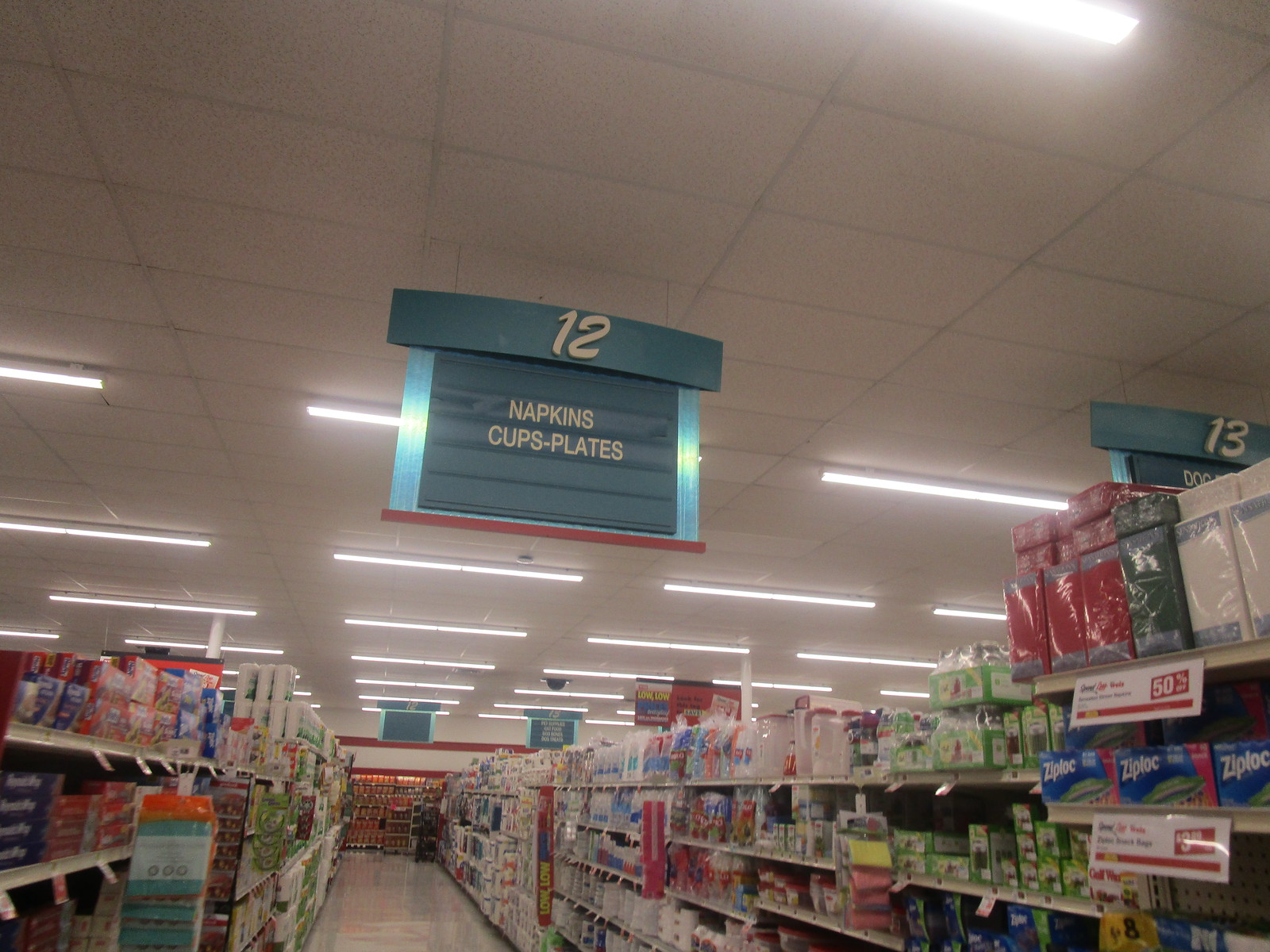This is a square color photograph of the inside of a supermarket aisle focused on paper goods. The white drop ceiling features long, fluorescent lamps arranged in parallel, extending towards the back of the room. Hanging from the ceiling by two black strings is a green sign indicating Aisle 12, which is primarily dedicated to "napkins, cups, and plates," with the text in white. This sign has a dark blue background with light blue accents on the sides and a distinct red line at the bottom. 

To the right, the shelves display an array of products, including Ziploc bags with a visible price tag of $3.99, as well as various types of napkins and plastic bags. Near the lower right corner, there's a prominently placed sticker indicating a 50% discount. The left side of the aisle features items such as aluminum foil and cling wrap. A glimpse of refrigerated drinks can be seen at the far end.

In the top right corner, another sign for Aisle 13 is partially visible, matching the color scheme of the Aisle 12 sign but obscured by the products on display. The shelves on the left also contain a mix of brightly colored packages, including green, red, blue, and orange items. The photograph captures the detailed organization and variety of products within this specific supermarket aisle.